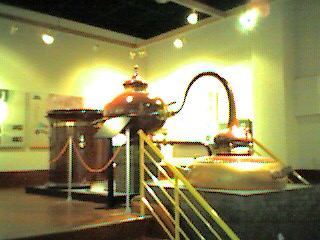This image captures a dimly lit museum exhibit featuring an intricate machine against a black background. Central to the photograph is a complex contraption, prominently displaying a large, round vat with a black top situated on a square, gray concrete platform. Attached to this vat is a hose that loops to the right before descending into another cylindrical component with a brass base.

Flanking the exhibit is a yellow stairwell with a safety railing, which might be part of an elevated platform in the room. The walls are painted yellow, contributing to the room's warm tone and enclosing the space, which appears to have decorative elements, possibly square paintings or images, hung and illuminated against the black ceiling. The scene is cordoned off with ropes and metal bars, preventing visitors from crossing into the exhibit space.

Overhead, lighting fixtures hang from the ceiling, casting light onto the various components of the machine. The room, devoid of people, exudes an industrial yet orderly atmosphere, with clear demarcations and an intentional exhibition layout.